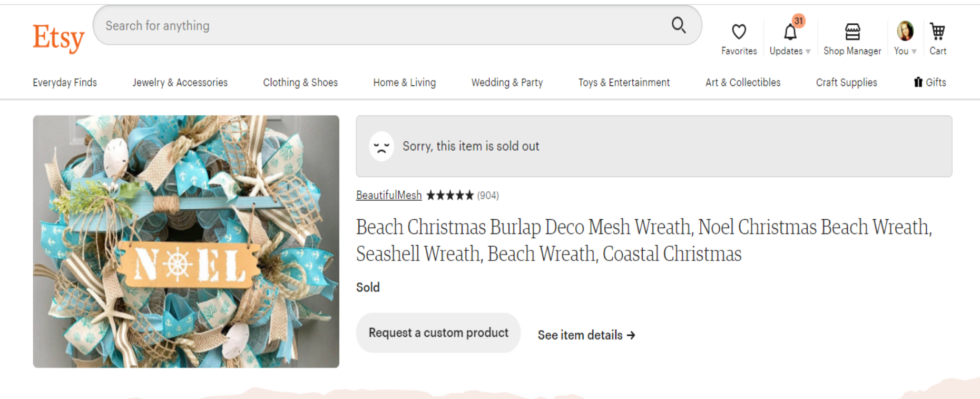Here is a cleaned-up and highly detailed caption for the image described:

---

The image displays a webpage from Etsy, highlighted by the Etsy logo in the upper left corner, colored in orange. To its right is a prominently placed gray search bar with the placeholder text "Search for anything," accompanied by a magnifying glass icon on the far right side. Adjacent to the search bar are navigation options: "Favorites," "Updates" with an orange circle containing the number 31, "Shop Manager," "You," and "Cart."

Beneath this, stretching across the top, is a category menu starting from the left with options for "Everyday Finds," "Jewelry & Accessories," "Clothing & Shoes," "Home & Living," "Wedding & Party," "Toys & Entertainment," "Art & Collectibles," "Craft Supplies," and "Gifts." A horizontal gray line separates this menu from the content below.

The main focus of the page is on the left, featuring an intricately designed wreath. The wreath comprises light blue ribbons, white starfish, and shells, with what appears to be jute ribbon resembling a fishing net. A paddle adorns the wreath, inscribed with the word "Noel." The product is labeled as "Beach Christmas Burlap Deco Mesh Wreath, Noel Christmas Beach Wreath, Seashells Wreath, Wreath Beach Wreath, Coastal Christmas," and is marked as sold. Two buttons are displayed: “Request a custom product” and “See item details.”

Above this wreath description, a gray bar with a frowning emoji indicates: "Sorry, this item is sold out."

---